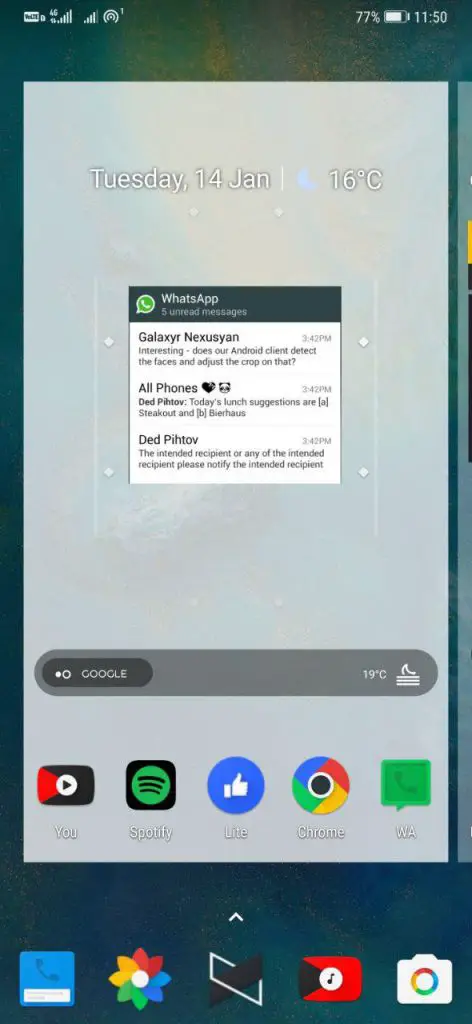The image is a detailed screenshot of a smartphone home screen. The background showcases a blend of grayish-green and blue hues, lending a subtle, serene aesthetic.

In the upper right corner, the time is displayed as 11:50, accompanied by a battery icon indicating a 77% charge. On the upper left, icons for the wireless connection are visible.

Dominating the center of the screen is a large, light silver-gray vertical rectangle. Inside it, there's a white box with a green top border, prominently featuring the WhatsApp logo, a green circle with a white phone symbol. Below this, the text reads "Galaxy N-E-X-U-S-Y-A-N," with smaller, unreadable fonts underneath.

Under this rectangle, there's a light gray rounded rectangle with "Google" written in white on the left side. This is followed by app icons including Spotify (green and black), the Facebook like button, Chrome, and another unidentified green app.

Lower on the screen against a darker background, additional icons are visible. These include an icon resembling the back of a credit card, one that looks like a colorful flower, two rectangles, a red square with a white circle and a black musical note, and a white camera icon.